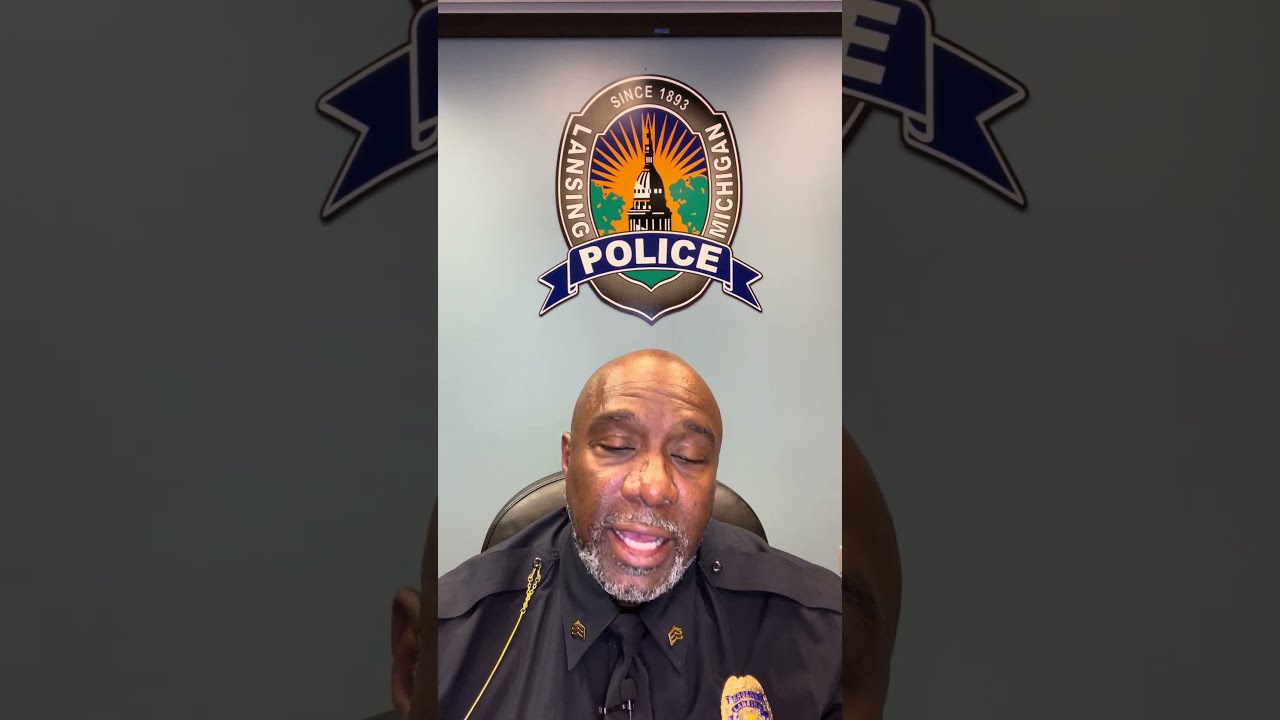A black man, bald with a prominent nose, is seated facing forward on a high-backed brown leather chair with the backrest reaching up to his neck. He has a goatee and a beard with streaks of gray and black, and his mouth is slightly open, revealing his bottom row of teeth. Dressed in a full black police uniform complete with a black shirt, black tie, and a distinctive cape-like accessory, the uniform features gold-colored emblems on the collar and a yellow cord hanging from the cape on the left side. Prominently displayed on his right chest is a gold police badge with blue lettering. 

Above him, the emblem of the Lansing, Michigan Police Department is prominently displayed. It features a banner at the bottom with a blue background and the word "POLICE" in all capital letters. The emblem itself is oval-shaped and enclosed in a brown circle, with "LANSING" on the left side, "MICHIGAN" on the right, and "SINCE 1893" across the top. Inside the emblem is a drawing of a domed building, with the sun shining from behind it and flanked by green leaves. The background of the wall behind the man is gray, with a black line running across the top. The left and right borders of the image contain enlarged, grayed-out elements of the main police emblem, providing a framed effect for the central portrayal of the officer.